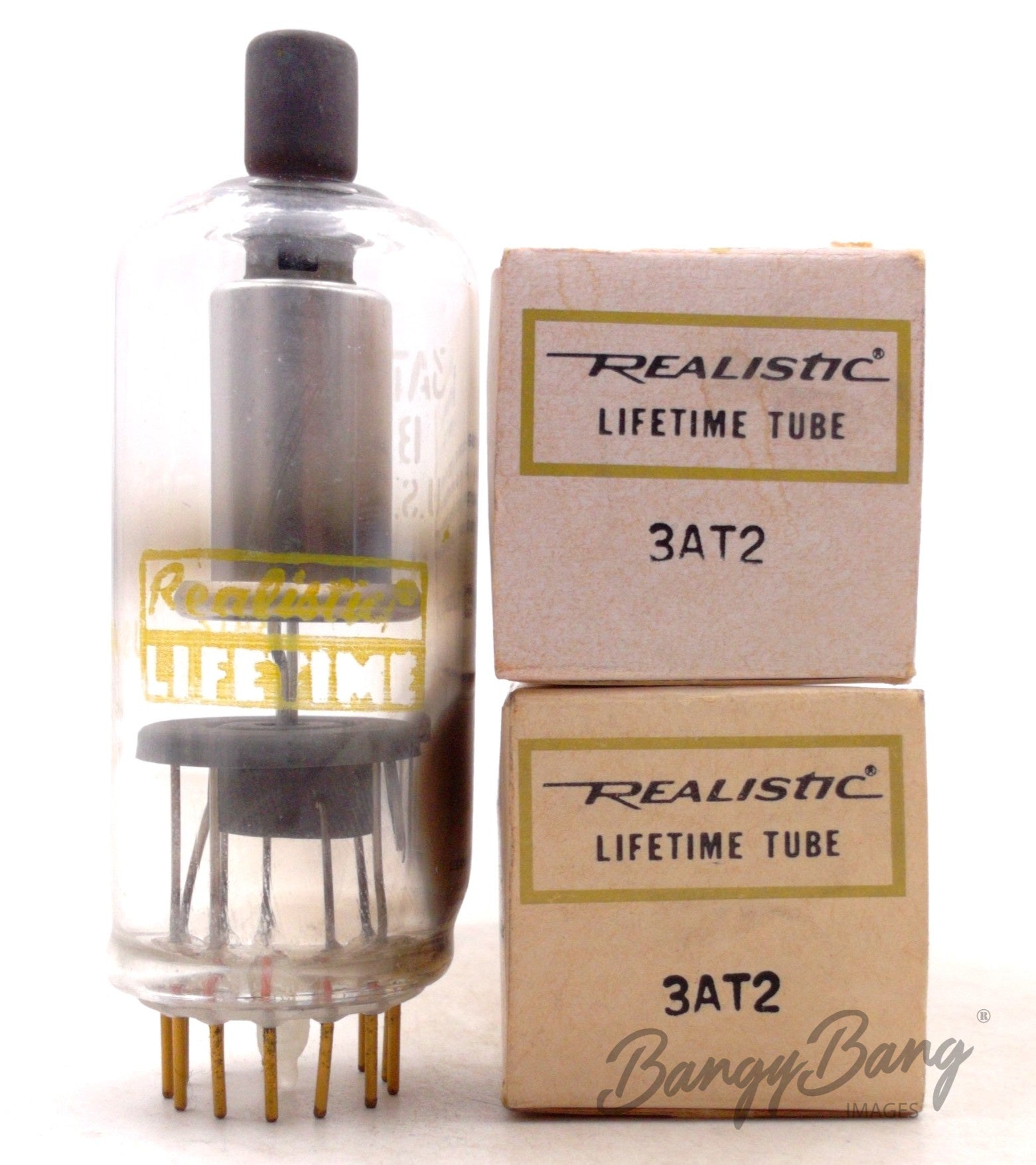The image showcases a vintage product arrangement against a white background. On the right-hand side, there are two peach-pink boxes labeled "Realistic Lifetime Tube," each marked with the model number 3AT2. Below the boxes, there is a light gray watermark that reads "Bangy Bang Image." To the left, a glass canister with a black top and metallic interior is prominently displayed, featuring the text "Realistic Lifetime" in yellow on its surface. The canister appears to contain a light bulb or tube, characterized by evident burn marks, suggesting it has been partially used. The overall setup is nostalgic, hinting at designs from the 1960s or 1970s, and the items rest on a pale pink table or counter. Green borders accentuate the box’s design, and the aesthetic is distinctly old-fashioned compared to modern light bulbs.